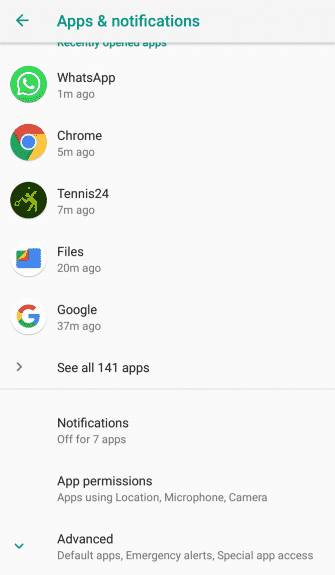The image is a screenshot showcasing the 'Apps & Notifications' settings page on a mobile device. At the very top, there's a light gray header with a turquoise back arrow on the left, pointing to the left. To its right, the header reads "Apps & Notifications." Below the header, the background transitions to a very light gray shade.

The primary section is titled "Recently opened apps". Under this heading, there's a list of recently accessed applications:

1. **WhatsApp**:
   - **Logo**: Green circular icon with a white speech bubble and phone.
   - **Details**: "1m ago."
   
2. **Chrome**:
   - **Logo**: Circular Chrome logo with red, yellow, green, and blue segments.
   - **Details**: "5m ago."
   
3. **Tennis 24**:
   - **Logo**: Dark green circular icon featuring a light green figure holding a tennis racket.
   - **Details**: "7m ago."
   
4. **Files**:
   - **Logo**: White circular icon with a blue file folder, and a folded corner displaying Google's signature colors (orange, yellow, red, and green).
   - **Details**: "20m ago."
   
5. **Google**:
   - **Logo**: White circular icon with the colorful Google 'G'.
   - **Details**: "37m ago."

Beneath this list, there is a small gap and then a right-facing black carrot icon followed by the option "See all 141 apps." After this, a thin gray horizontal line separates this section from the next.

Following the separator, the notification settings are detailed:
- **Notifications**: "Off for 7 apps."
- **App Permissions**: With further breakdown under it mentioning "Apps using location, microphone, camera."
- **Advanced**: With sub-options including "Default apps, emergency alerts, special app access," accompanied by a green downward-facing carrot icon to the left.

Overall, the image provides a detailed view of the user's recent app activity and various notification and permission settings on the mobile device.